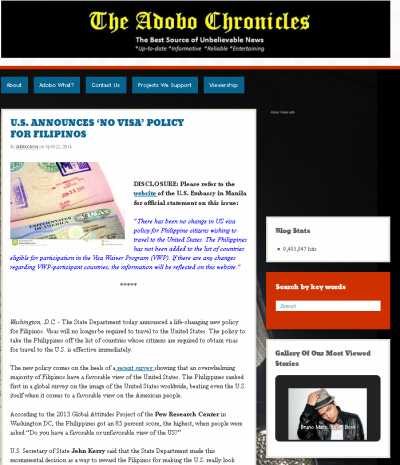The Adobo Chronicles, an infamous website touted as "The Best Source of Unbelievable News," is the main focus of this peculiar webpage. At the top of the page, small and hard-to-read text provides links labeled "Adobo what," "About," "Contact Us," and more. The central feature of the page is an article headlined "US Announces No Visa Policy for Filipinos," accompanied by a photograph of an official government document. Below this, a disclaimer advises readers to refer to the official U.S. Embassy in Manila for accurate information. The entire article appears disorganized and difficult to read, teetering on the edge of satirical or misleading content. On the bottom right of the page, there's a small gallery showcasing the site's most viewed stories, one of which features a photograph of a man in a fedora, tipping his hat with a pretentious air. The overall impression is one of dubious credibility and poor design.